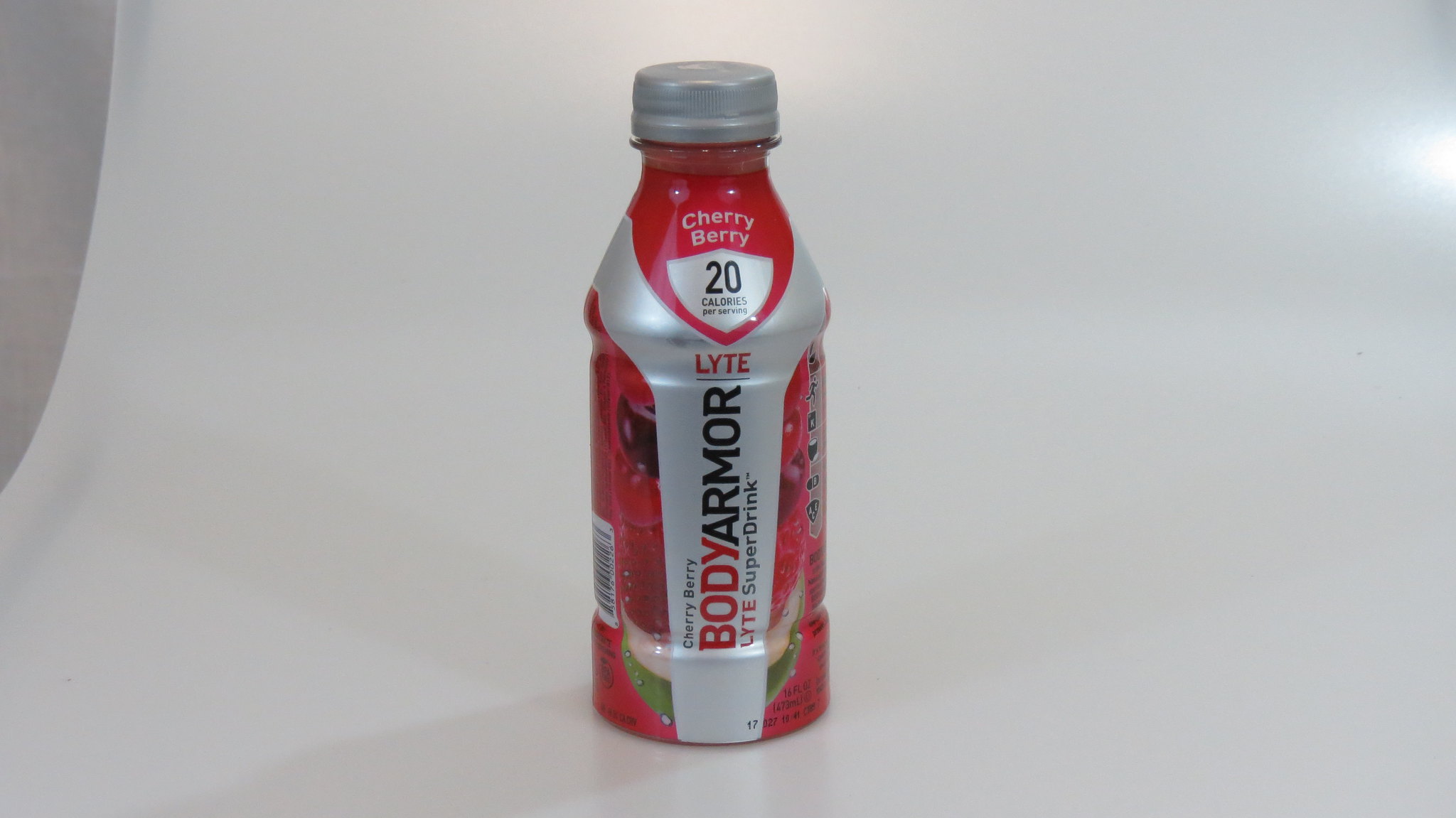In this horizontally rectangular image, the background transitions from white to off-white, creating a clean and minimalistic setting. In the upper right corner, a bright glare appears at the edge. Positioned centrally is a short plastic drink bottle, capped with a silver lid. The bottle's label features a striking design reminiscent of a silver tie, which extends from each side towards the center. At the top center of the label, where the tie splits, a red area prominently displays the text "Cherry Berry." The tie itself contains vertical text that must be read from bottom to top and includes the phrases "Cherry Berry," "Body Armor," "Light," and "Super Drink."